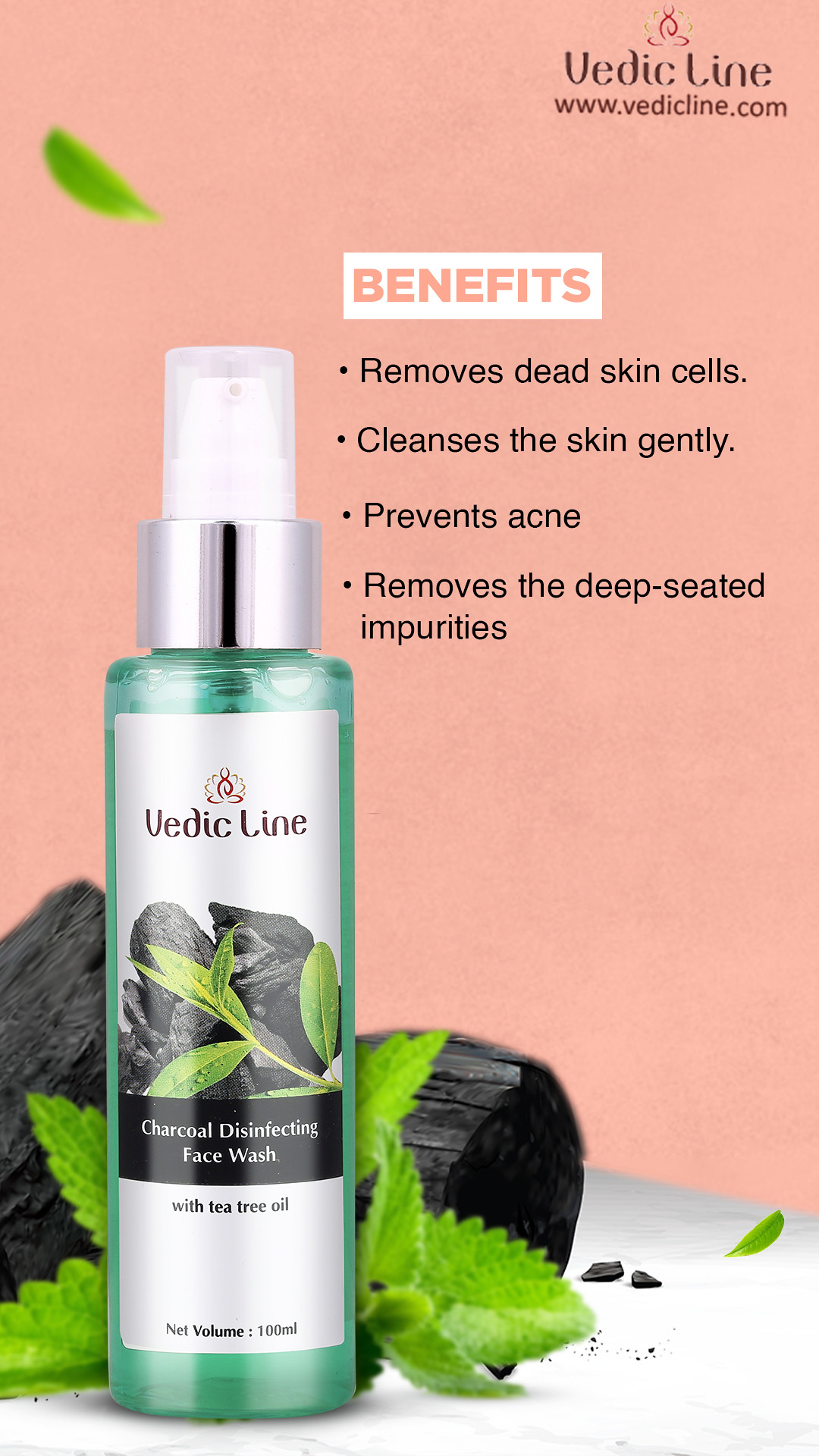The image is an advertisement for Vedic Line Charcoal Disinfecting Face Wash. The setting features a cylindrical green spray bottle with a white logo that says "Vedic Line," positioned in the lower left corner. The green bottle displays an image of black charcoal and green leaves. It has a yellow round section and a white cylindrical lid on top. Behind the bottle, there are more charcoal pieces and green leaves on a gray surface, all set against a pinkish-peach background.

In the upper right corner, the text "Vedic Line" and the website "www.VedicLine.com" are prominently displayed. Below this, a white rectangle with pink or peach “Benefits” text highlights four key features in black bullet points: "Removes Dead Skin Cells," "Cleanses the Skin Gently," "Prevents Acne," and "Removes the Deep-Seated Impurities." The overall design focuses on the product’s benefits with a clean layout, emphasizing the face wash bottle and its natural ingredients.